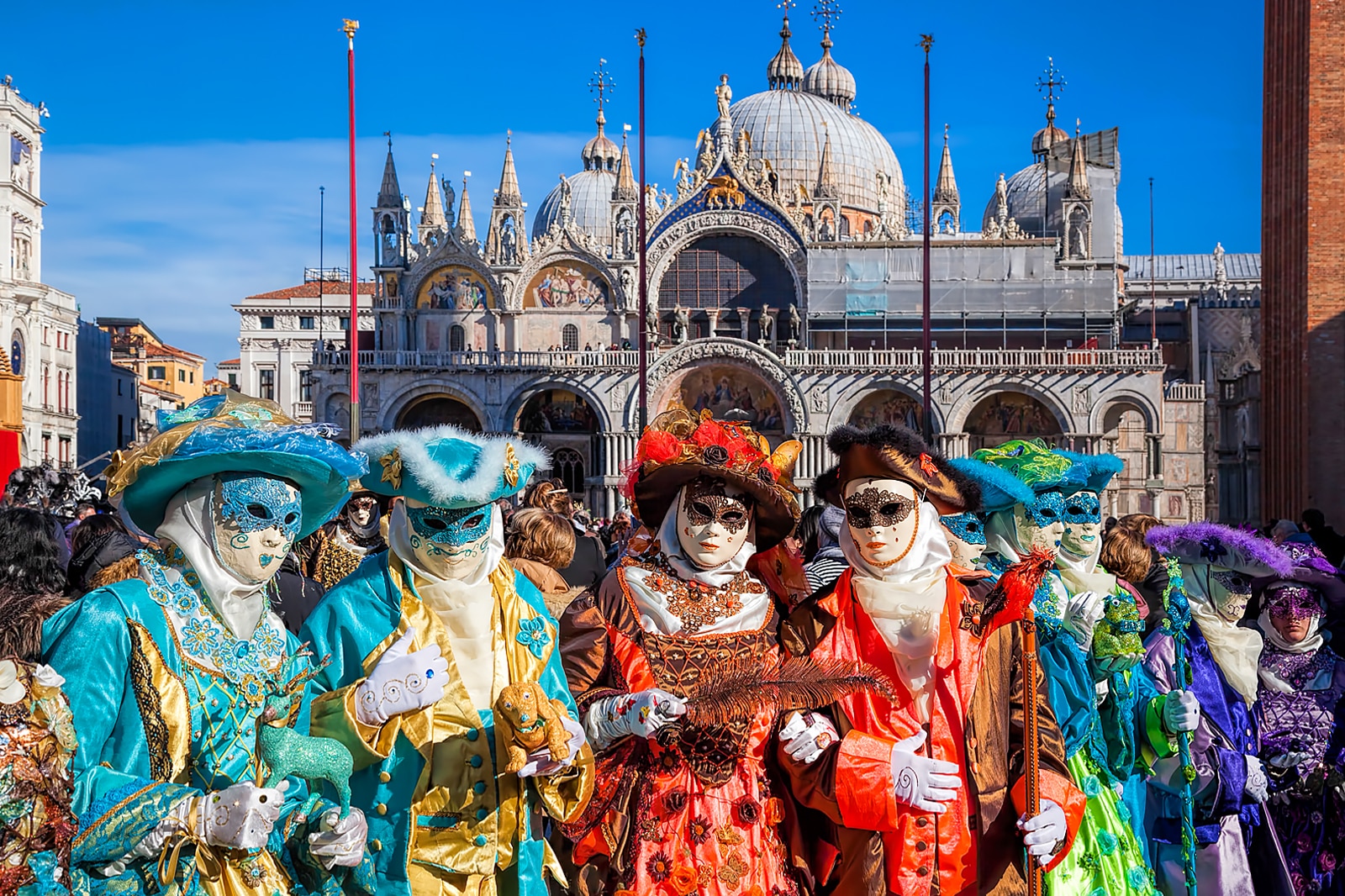In the image, the scene depicts an ornate, domed cathedral against a vibrant blue sky with some white clouds scattered below. The cathedral showcases intricate domes and spires, many topped with crosses and weather vanes. Below this majestic structure, a modern building stands out on the right, contrasting the historical architecture.

To the left of this, more city buildings are visible, including a brick building with a chimney. In the foreground, a group of elaborately dressed individuals in masks and costumes dominates the scene. The costumes are lavish, featuring vibrant blues, golds, purples, and reds, with intricate details such as white gloves, white vests, and feathered or fur-trimmed hats.

Among these people, specifics include individuals in matching blue hats with white feathery trim, blue and gold silk dresses, and blue masks with white eye cutouts. Two women in red hats adorned with flowers and brown masks hold long feathers. Other costumes vary with colors such as blue, green, and purple, each maintaining an ornate style.

Overall, the image beautifully blends historic and modern elements with a festive, almost surreal atmosphere due to the masked and costumed figures in the foreground.